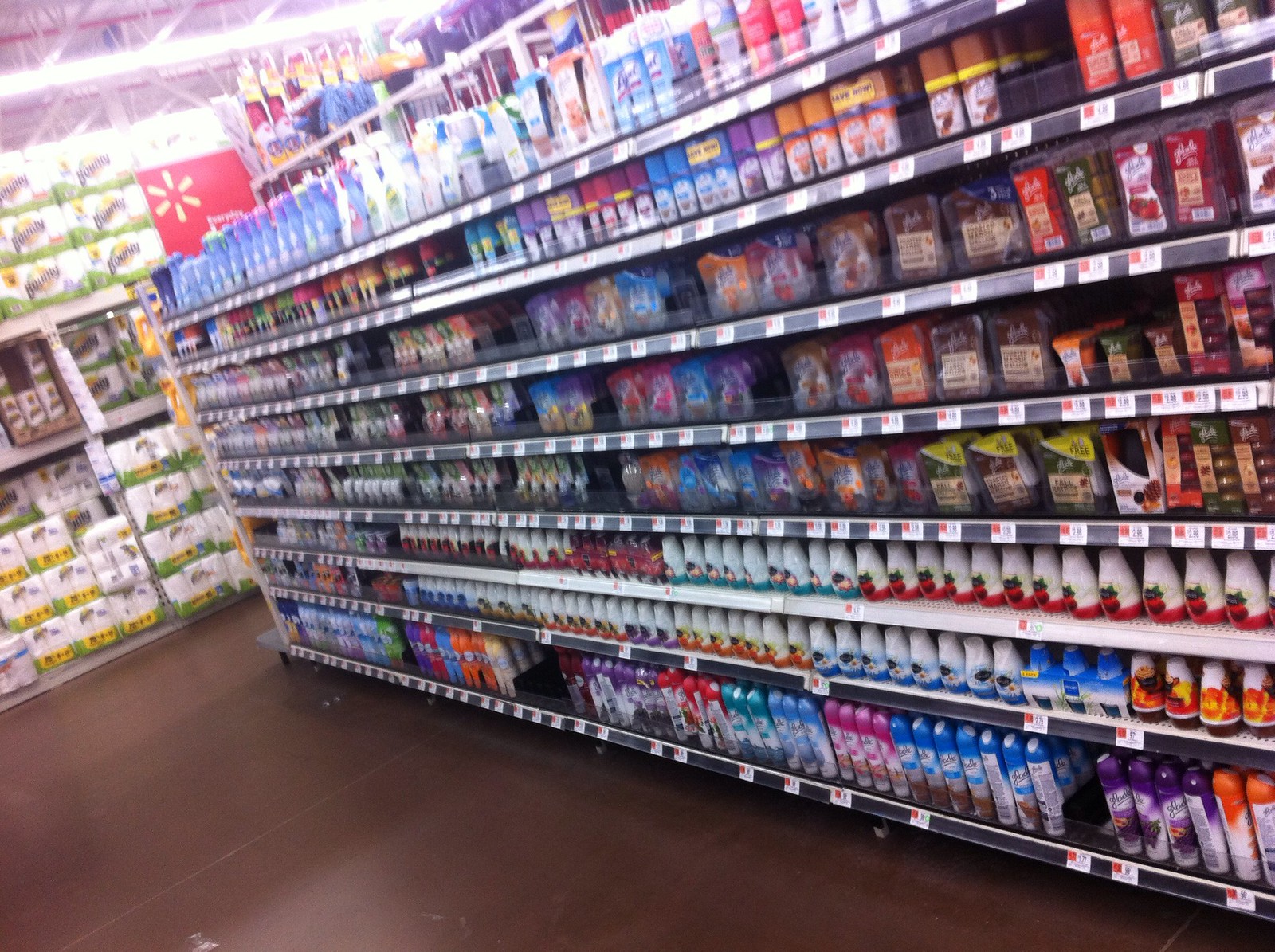In this color photograph taken indoors, we are presented with a detailed view of a store aisle dedicated to cleaning supplies. The floor of the store is dark brown, providing a rich contrast to the neatly arranged rows of horizontal shelves. Most prominent on the top shelf are an assortment of Lysol spray cans, iconic for their vibrant blue, green, and yellow labels. Adjacent and below, we see a variety of air fresheners and potentially some potpourri, adding a splash of fragrance options to the visual lineup. Each product shelf is equipped with long metal fronts adorned with small white square price tags, ensuring customers can easily identify product costs. In the background, additional shelves brimming with Bounty paper towels are visible, indicating a well-stocked and organized aisle designed to meet a range of household cleaning needs.